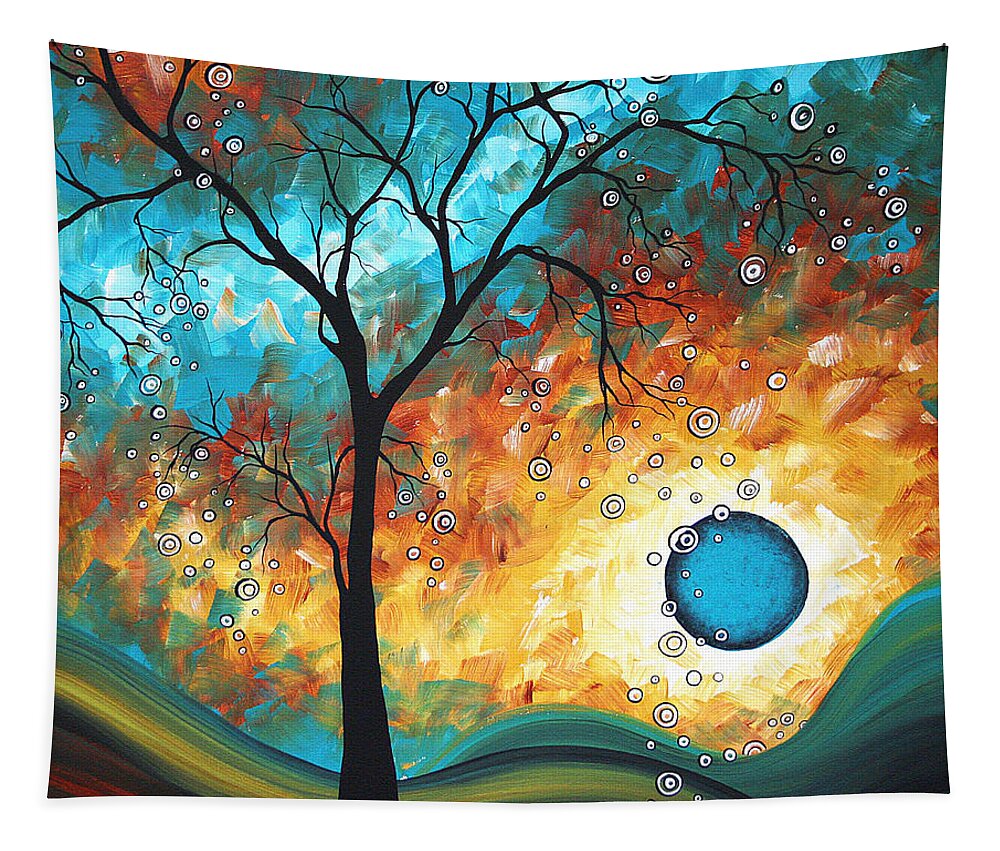The painting presents a single, barren tree with gnarled branches as the main focus, centrally positioned in the foreground. The tree is painted in stark black, creating a striking silhouette against an intricate, colorful background. Dominating the background is a vibrant red sunset, infused with rich shades of orange, yellow, and red, transitioning into a lighter blue sky at the very top. Superimposed on this vivid scene are numerous tiny white circles, which could suggest snow or simply be a magical, otherworldly element. Amidst this dreamy landscape, a blue orb, possibly depicting a planet or moon, adds a touch of fantasy. The ground at the base of the painting is formed by undulating, wavy lines in an array of colors, including green, yellow, red, teal, aqua, gold, mustard, black, and purple, representing rolling hills or layered terrain. The entire composition evokes a mystical, nature-inspired scene that merges elements of reality with the fantastical.